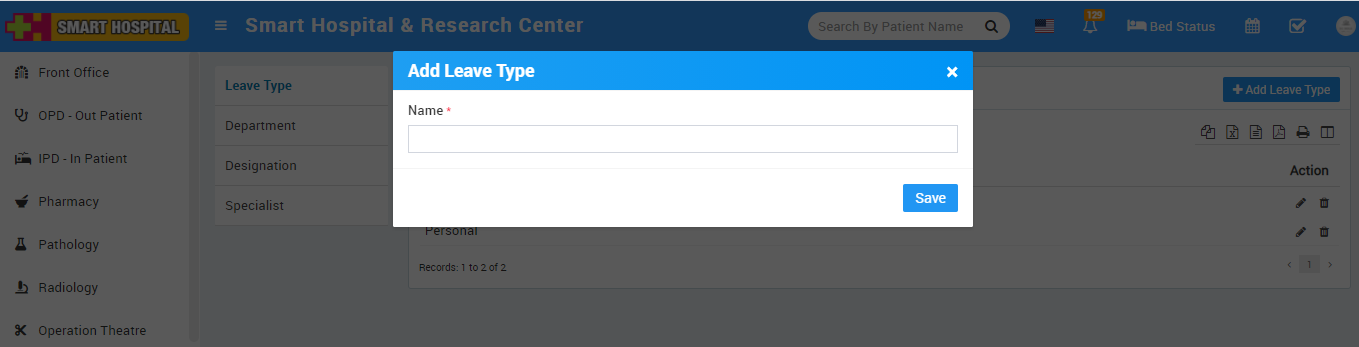The image features a partial screenshot of a website with a grayed-out background due to a prominent pop-up box in the center. The page header is visible despite the overlay. On the left side of the header is a yellow rectangle containing the text "Smart Hospital" in white letters outlined in black, accompanied by a red "X." Adjacent to this, the header stretches across the top with a blue border and the phrase "Smart Hospital and Research Center" written in white. To the right, a white search box is partially visible, along with other less discernible items.

The central focus of the image is the pop-up box, which is rectangular in shape. The top section of the pop-up is blue and contains the text "Add Leave Type" in white font. The main body of the pop-up is white, featuring a label on the left side that reads "Name" next to an outlined box intended for entering a name. In the lower right-hand corner of the pop-up is a small blue rectangle with the word "Save" written in white.